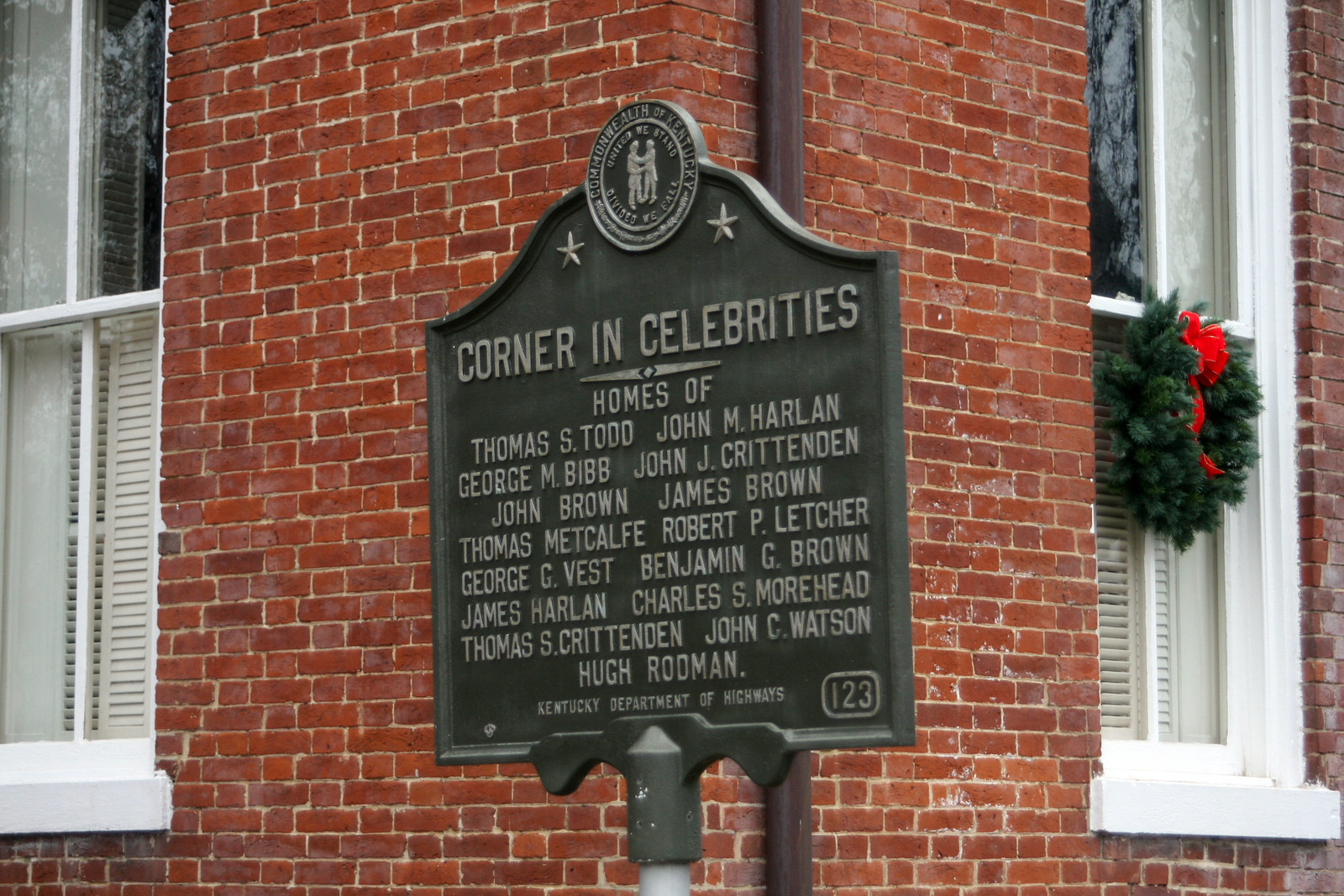This image captures an older looking metal sign positioned in front of a brick building with white wooden window panes. The sign, predominantly green with white lettering, lists significant historical figures, stating: "Corner in Celebrities. Homes of Thomas S. Todd, John M. Harlan, George M. Bibb, John J. Crittenden, John Brown, James Brown, Thomas Metcalfe, Robert P. Letcher, George G. Vest, Benjamin G. Brown, James Harlan, Charles S. Moorhead, Thomas S. Crittenden, John C. Watson, and Hugh Rodman. Kentucky Department of Highways 123." The brick building in the background features various shades of red and brown, with two large windows. The window on the right includes a festive wreath adorned with a red ribbon, adding a splash of green to the composition. Overall, the photo appears to have been taken casually, capturing the scene in natural light with colors ranging from light and dark gray to white, and multiple tones of red and brown.